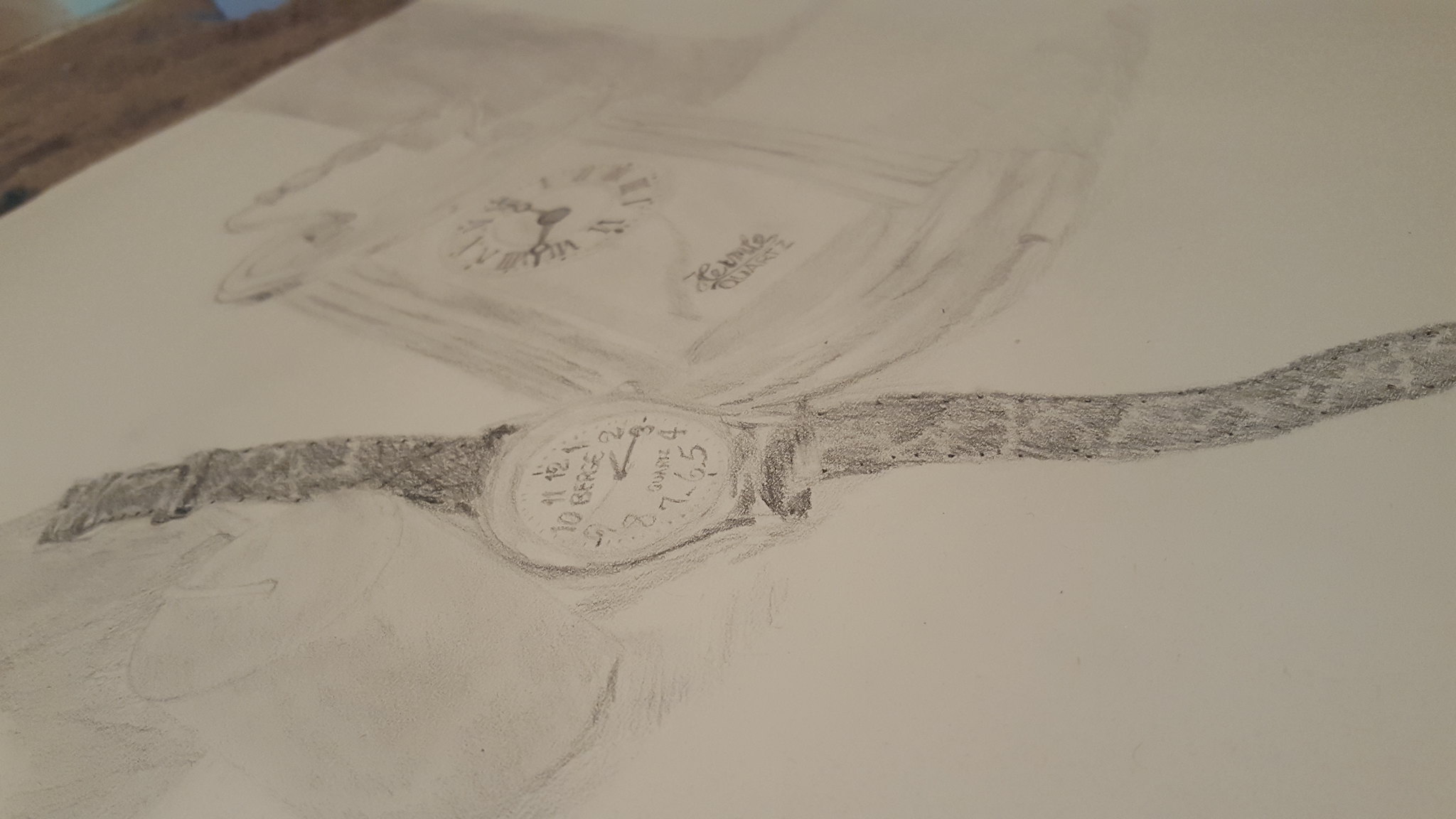This is a photograph of a meticulously hand-drawn illustration, primarily executed in pencil, showcasing two distinct timepieces. The focal point of the drawing is a wristwatch with an intricately designed, delicate wristband adorned with subtle white and gray patterns. The clock face of the wristwatch is exquisitely rendered, with soft gray numbers and darker, finely etched hands that add depth and emphasis to its elegant appearance. Adjacent to the wristwatch, there is a faintly sketched outline of a grandfather clock, characterized by its tall and imposing structure. The clock displays Roman numerals on its face, and the lower section features cursive writing, though the exact text remains indeterminate due to its faintness. The white paper background of the image contains some stray pencil marks, adding a touch of authenticity and the artist’s process to the composition.